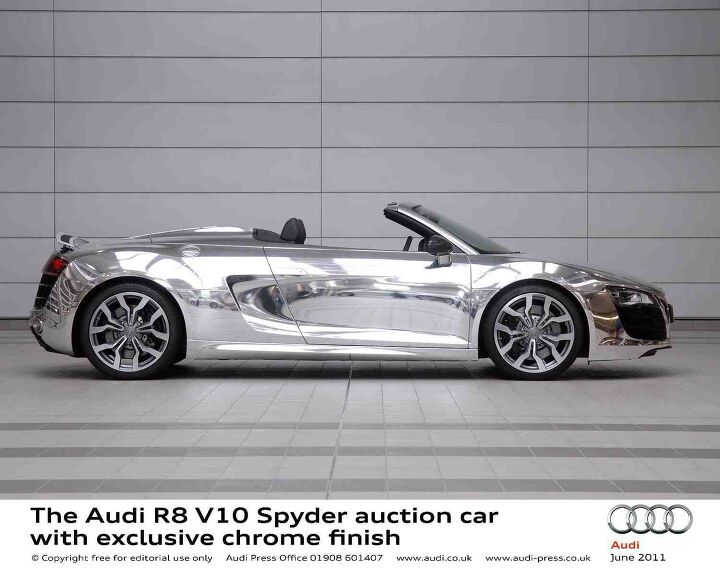The image showcases an Audi R8 V10 Spyder, a striking convertible car with an exclusive chrome finish, giving it a superficially shiny, mirror-like appearance. The car dominates the foreground, positioned horizontally to highlight its sleek, silver metallic body that reflects its surroundings. It rests on a gray tiled floor, which features three distinct thicker gray stripes toward the front, and is backed by a gray paneled wall resembling a high-end garage or showroom. Notable text at the bottom of the image reads, "Audi R8 V10 Spyder Auction Car with Exclusive Chrome Finish," alongside the Audi logo and additional details: "Audi June 2011" and information indicating it's copyright-free for editorial use, provided by the Audi press office with accompanying website URLs.